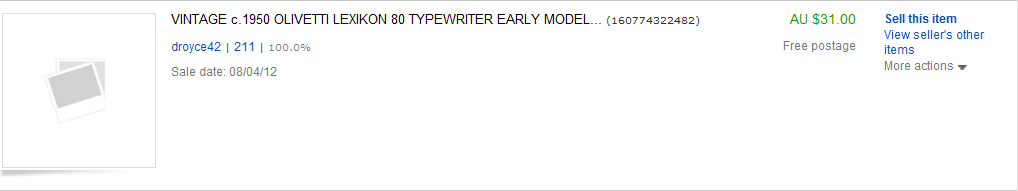This image is a cropped screenshot of an email listing for a vintage typewriter. The rectangular screenshot highlights an item titled "Vintage 1950 Olivetti Lexicon 80 Typewriter Early Model" with an identification number next to it in parentheses. Below the title, the seller's name, "choice42," appears in blue, accompanied by their sales statistics showing they have made 211 sales, boasting a perfect 100% positive rating.

The item was sold on August 4th, 2012. On the left side of the listing, there is a placeholder for an image of the typewriter, represented by a Polaroid icon, indicating that an actual image could be displayed there, though it is currently blank.

The sale price is listed in Australian currency (AU) as $31, with the added benefit of free postage. Additional text on the listing provides options for viewers, including "Sell this item" for those who have a similar item to sell, and "View seller's other items" to explore more listings from the same seller.